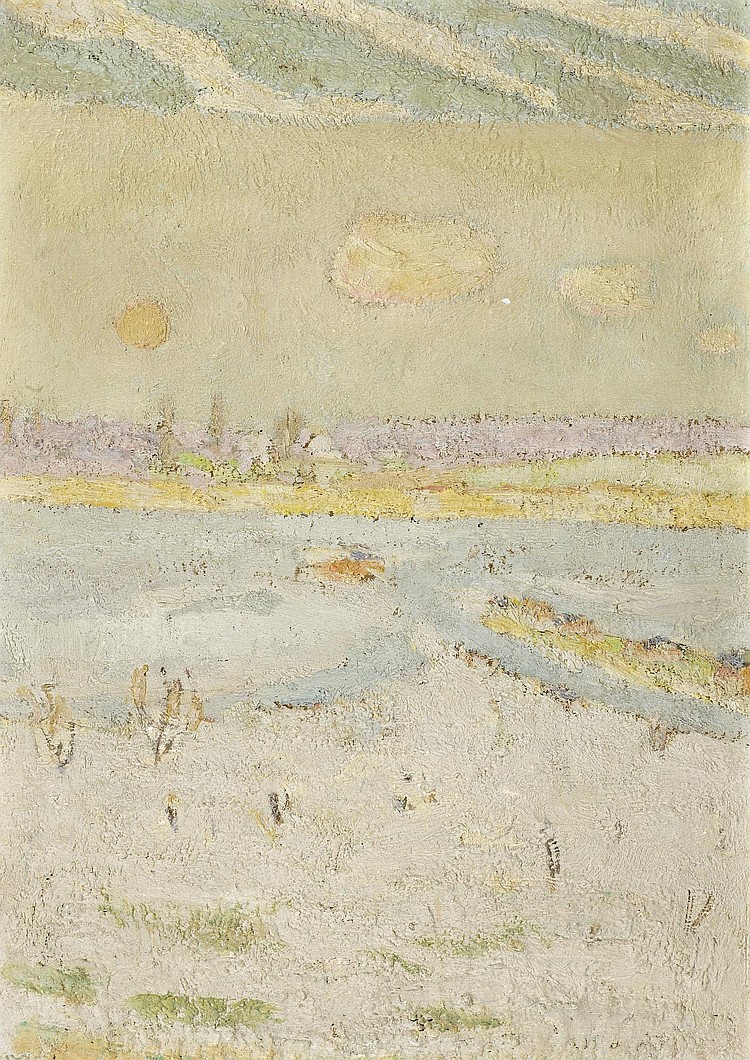This abstract painting captures an indistinct outdoor setting, possibly depicting a river during daytime. The palette comprises extremely light and soft tones, including bone, pale blue, pale yellow, light pink, cream, and smoky gray. The scene unfolds with a very light blue river flowing along a creek bed, adorned with a white frosting-like texture on the water surface. Intriguing orange elements punctuate the center of the stream. At the river's edge, specks of grass and dead weeds emerge, while a streak of green suggests the presence of an alligator moving from right to left. The riverbanks feature brown and yellow strips with dead leaves and weeds, topped with light purple ground.

On the opposite bank, a smooth, grayish mountain ascends, adorned with light orange circles and streaks reminiscent of irrigated farm rows. The horizon consists of gray bands with orange cloud-like formations, transitioning upward to a blue sky streaked with diagonal white clouds. The overall impression is abstract, with layers of color blending together to suggest an impressionistic interpretation of a serene, natural landscape.